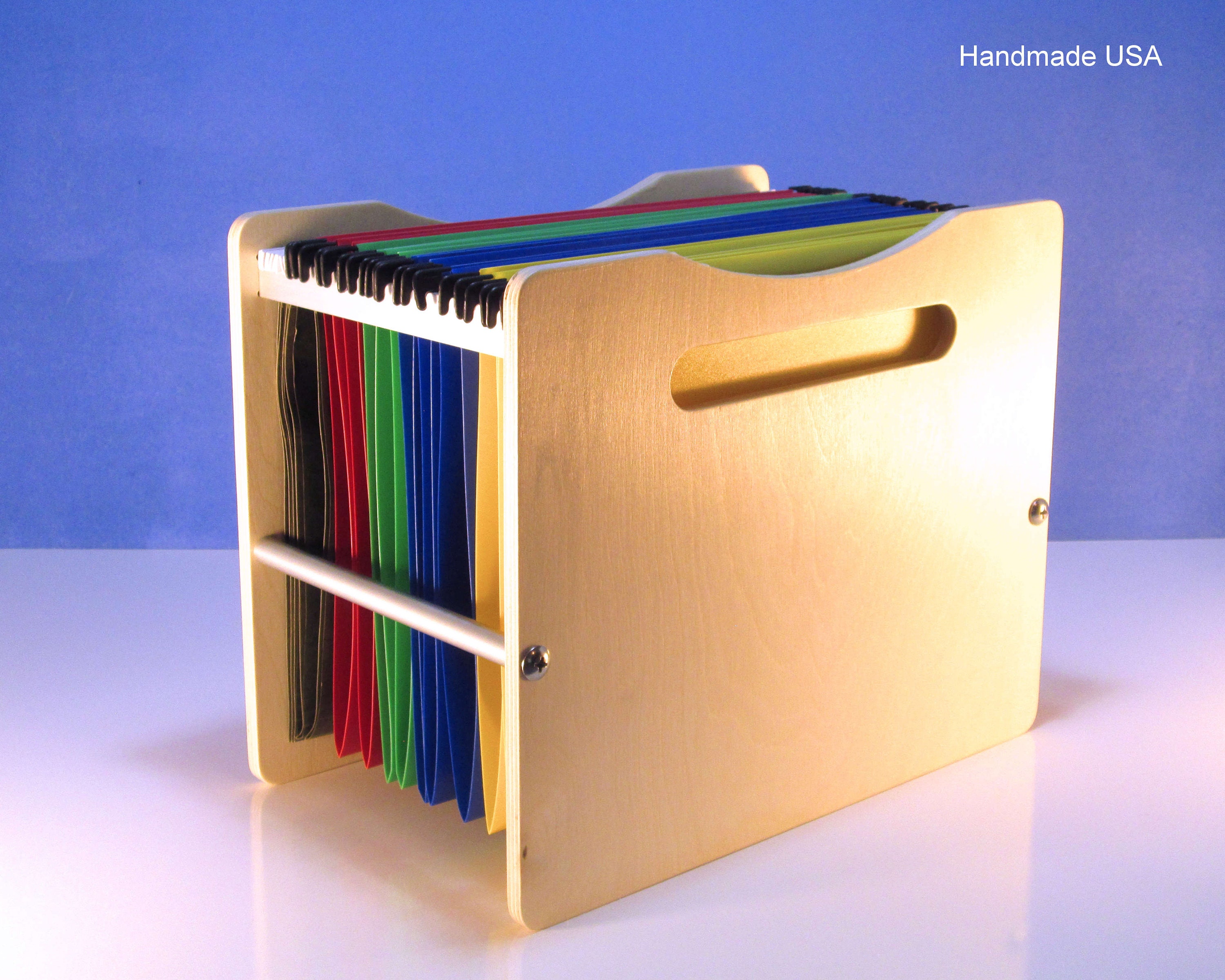This horizontally aligned photograph features a composition divided into two distinct halves: the upper half, a royal blue background, and the lower half, a shiny white surface that reflects its surroundings. The upper right corner of the photograph contains white text reading "Handmade USA" in Comic Sans font, suggesting it could be an advertisement from the past 15 years.

In the foreground, the central object is a meticulously crafted wooden file holder, likely made from teak or a similar tan wood. This file holder has two identical solid sides, each with a large, shallow arc cut into the top, resembling a handle. The wood has a bare, light tan finish, appearing well-sanded and smooth. Horizontal metal rods, one near the top and another about 3 cm below it, connect these solid sides. These rods are slightly diagonal in the image, higher on the left side, and the lower rod features visible bolts securing it.

The holder contains ten hanging file folders suspended from these rods. Organized from left to right, the folders are black, red, green, blue, and yellow, with two of each color. The glossy white surface beneath the holder reflects light and casts subtle shadows to the upper left, bottom left, and upper right, adding depth to the scene.

In the middle far right of the lower background, a pinkish reflection suggests the presence of a light source, while a white light in the far left corner transitions into a blue hue, reflecting the upper blue background. The overall impression is one of precise craftsmanship and vibrant organization, set against a backdrop that amplifies the polished nature of the wooden file holder and its colorful contents.